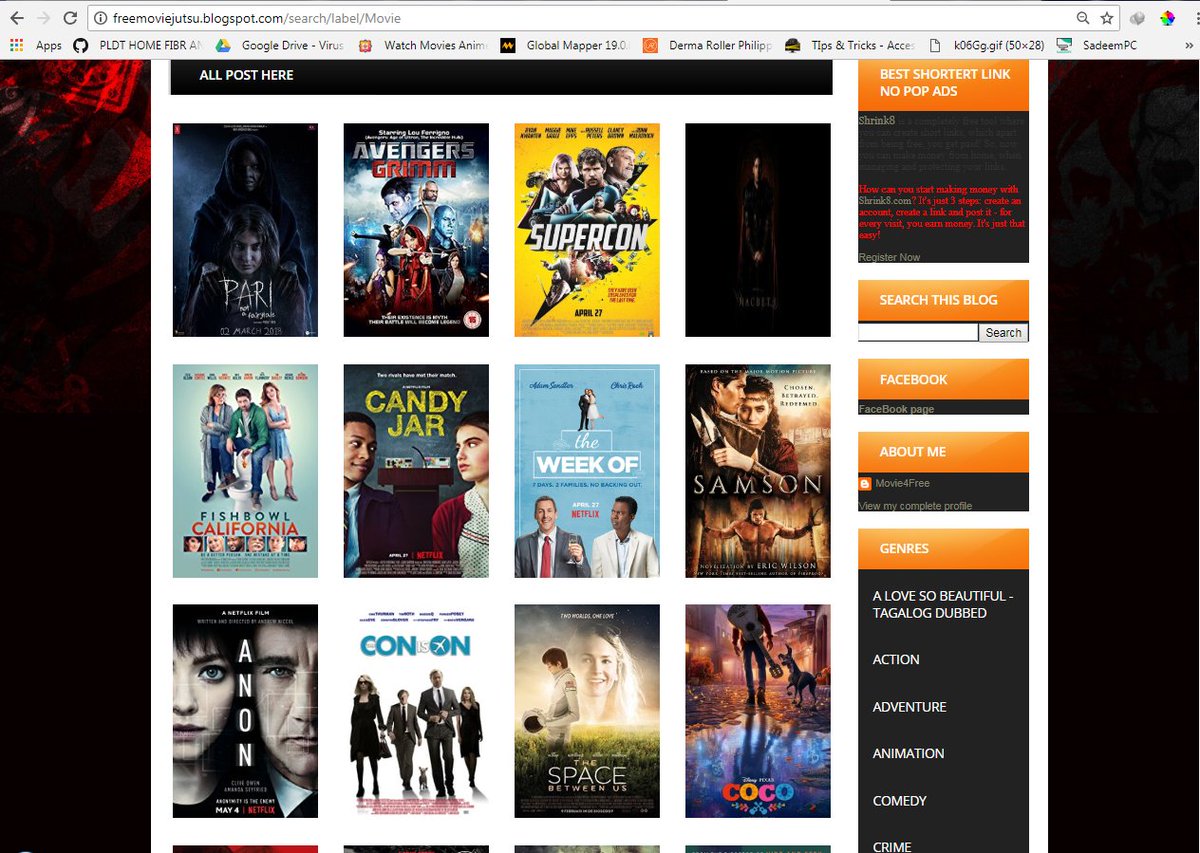**Detailed Caption:**

This is an image from the website freemoviejutsu.blogspot.com, which offers a variety of movies for free streaming. The top of the page features a search bar with several links reading: "Google Drive watch movies," "global map," "a derma roller tips and tricks," and another unspecified website. Additionally, "sardine PC" is mentioned alongside the top navigation.

The layout of the webpage includes two vertical black lines running from the top to the bottom margins on the left and right sides. The left margin is adorned with red, abstract designs. Below the search bar, there is a black box with the text "All posts here" spanning across the top.

The main section beneath this contains a series of movie cover images. The titles visible include "Perry," "One's Adventures," "Grim," and other titles with corresponding cover images. One cover appears predominantly black with an indistinct ghostly figure with dark, possibly reddish hair. Another cover shown features a fishbowl representing "California," alongside covers for "Candy Jar," "A Week Of," "Samson," "Anon," "Kanan," "Space," and "Cocoa." Further movie covers are visible but get cut off toward the bottom.

On the right sidebar, the text reads: "Best shortest link no pop ads," followed by clickable links labeled "Search the blog," "Facebook," "About me," and "Genres," all highlighted in orange. The list of movie genres visible includes "Action," "Adventure," "Animation," and "Comedy," but extends beyond the visible portion of the screen.